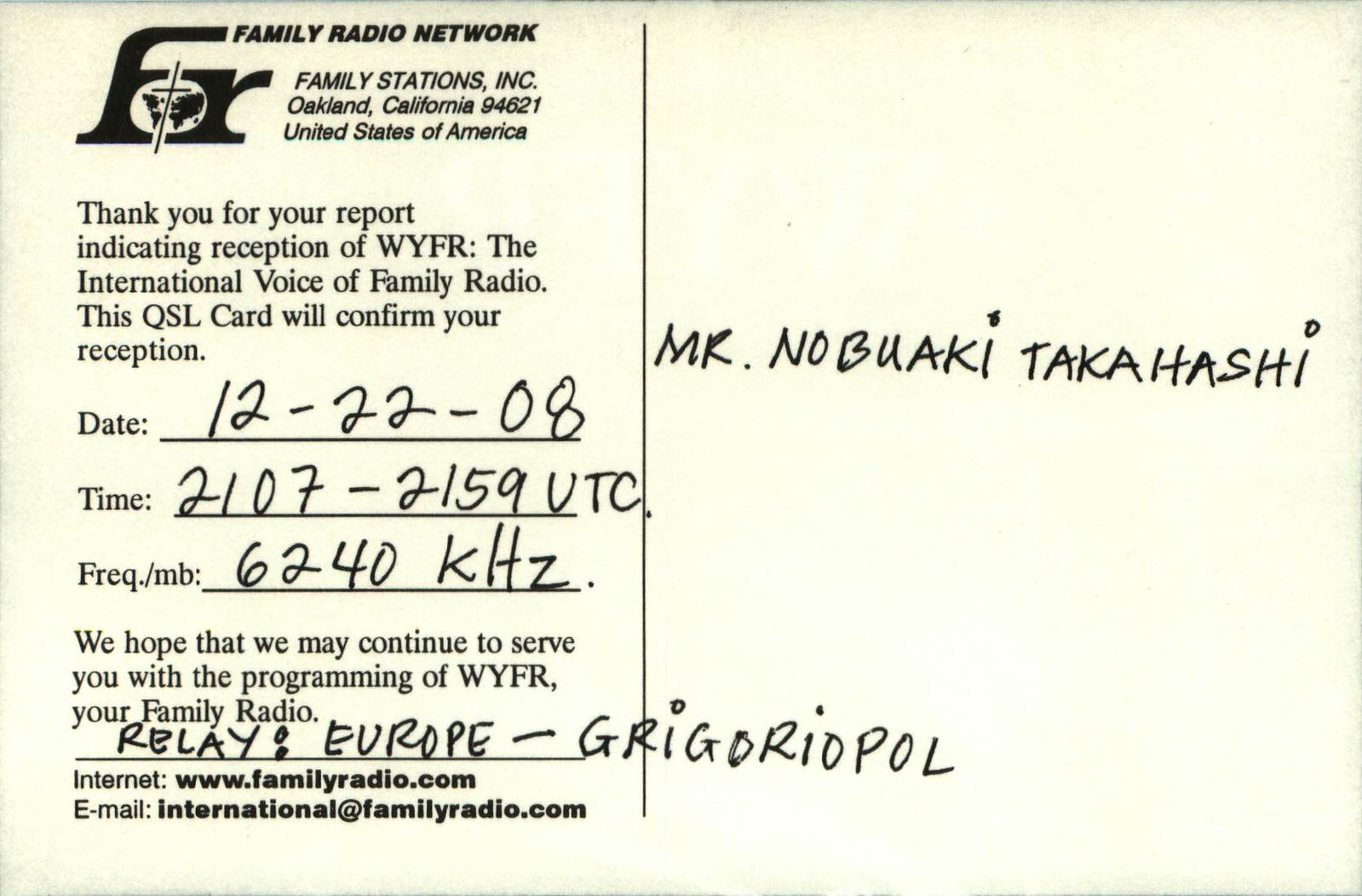This image displays the back of a QSL postcard from the Family Radio Network, Family Stations Incorporated, based in Oakland, California, 94621, United States. The card thanks the recipient, Mr. Nobuaki Takahashi, for his report confirming the reception of WYFR, the International Voice of Family Radio, on December 22, 2008. The report specifies the reception time as 21:07 to 21:59 UTC on the frequency of 6240 kHz (6.24 MHz). The message expresses hope to continue serving the recipient with WYFR programming, relayed in Europe by Gregorio Pol. Additionally, the postcard includes an internet website, www.familyradio.com, and an email address, international@familyradio.com.